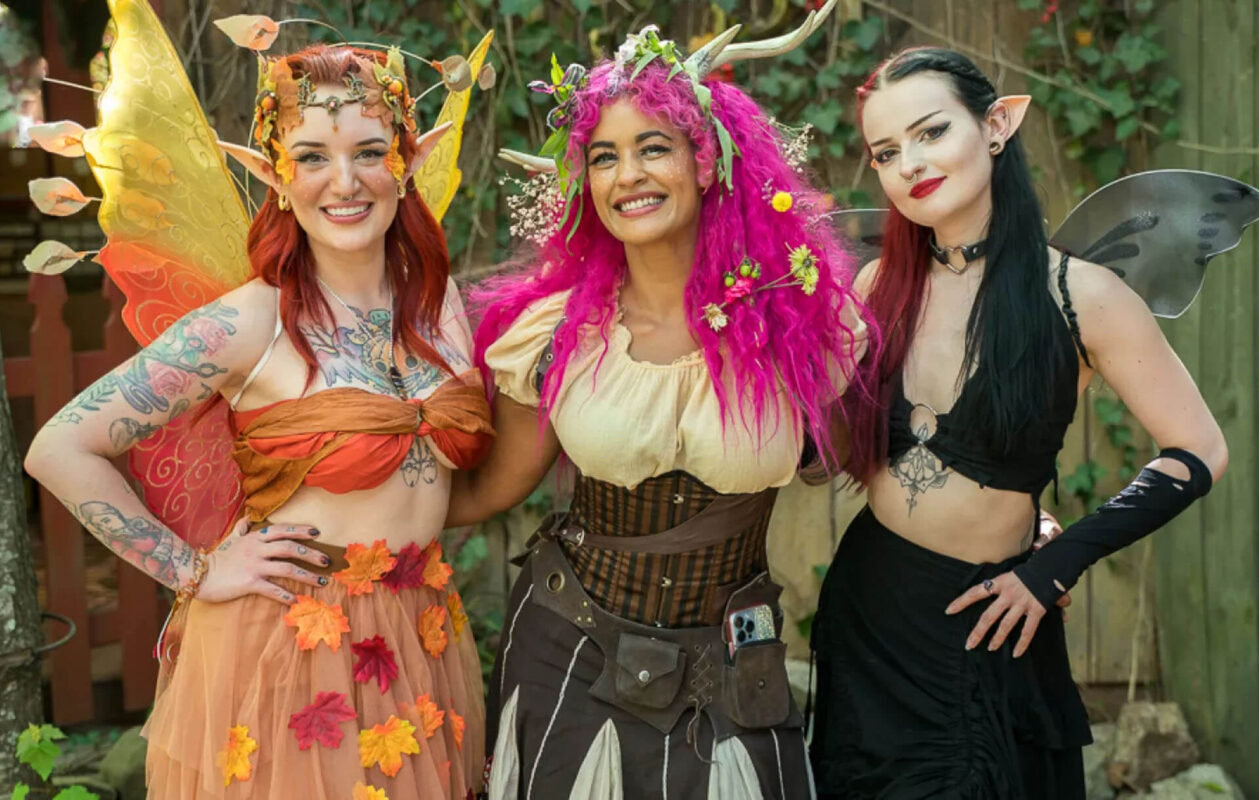The image features three women dressed as fantasy characters, standing closely together in front of a backdrop that includes a mix of brown and greenish fences covered with leafy vine bushes in varying shades of green, yellow, and reddish hues. At the bottom right, there's a cluster of white-gray rocks, while the bottom left features darker gray rocks surrounded by green leaves and topped with a red fence. The scene gives off a festive, possibly Halloween-themed vibe. 

The woman on the left wears elaborate yellow, red, and pinkish fairy wings, complemented by red hair and elf ears. Her attire includes a red and orange bra-like top, a pink skirt adorned with orange, yellow, and purple leaves, and visible tattoos in black, red, orange, and green hues.

The central figure sports purple hair decorated with yellow and red leaves. She has on an off-white top with a black corset featuring brown lines and a central brown strip, along with a brown belt equipped with a smartphone in one of its pockets. Her skirt is striped white and brown, and she accessorizes with white or tannish horns on her head.

The third woman, exuding a goth or emo fairy aesthetic, has half-red, half-black hair. She is adorned with a black leather choker with a silver heart, red lipstick, elbow-length black gloves with rips, a black top with a silver circle, a black tattoo on her stomach, and a black skirt. 

Together, they form a striking tableau of fantasy and fairy-tale inspired costumes, accentuated by the vibrant and varied backdrop.